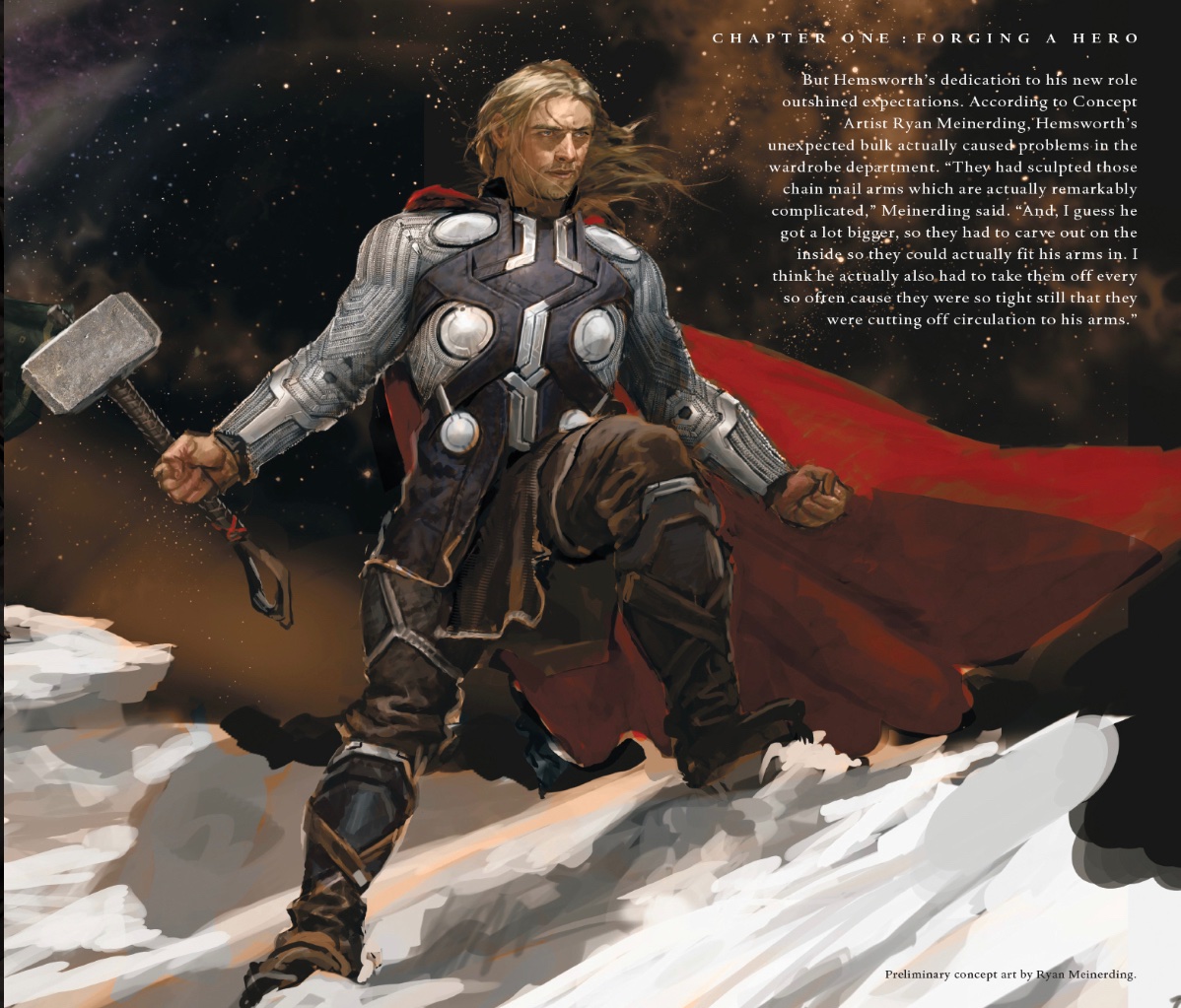This preliminary concept art by Ryan Meinerding showcases a Thor-like character, likely portraying Chris Hemsworth as Thor, standing heroically on a snowy mountain cliff top. Central to the image, Thor wields a silver hammer in his right hand, while his left hand is clenched into a fist. He is clad in intricate silver and black chest armor, complemented by brown and black pants and sturdy boots. A long, flowing red cape billows out to his right. The character has striking white skin, long blonde hair being swept by the breeze, and a light beard, embodying the iconic look of the Norse god. The backdrop of the scene is a mesmerizing starry night sky. In the upper right corner of the image, the text "Chapter 1: Forging a Hero" is displayed, highlighting the beginning of Thor’s journey. Accompanying the artwork is a caption detailing Hemsworth's significant physical transformation for the role. Concept artist Ryan Meinerding remarked that Hemsworth's unexpected increase in muscle mass presented challenges for the costume designers, particularly with the sculpted chainmail arms, which had to be modified internally to accommodate his bulk. Despite these adjustments, the tight fit of the costume often restricted circulation, necessitating periodic removal.